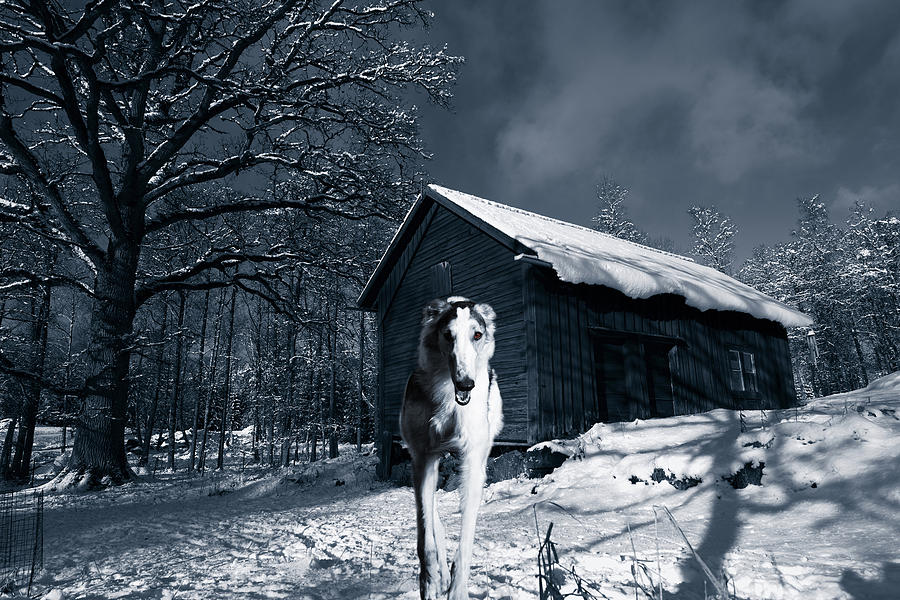In the image, a dog is positioned facing the camera, capturing the full view of its face, chest, and both front legs, with a glimpse of its back right leg visible. The backdrop features a snowy, slanted hillside, suggesting a small incline. Situated in the background, slightly to the right, is a one-story cabin with an A-frame roof, adorned with a layer of snow. The cabin is oriented towards the lower right of the frame, showcasing both its front and right sides. This cozy, snow-covered setting complements the dog’s poised and attentive stance, creating a picturesque and serene winter scene.